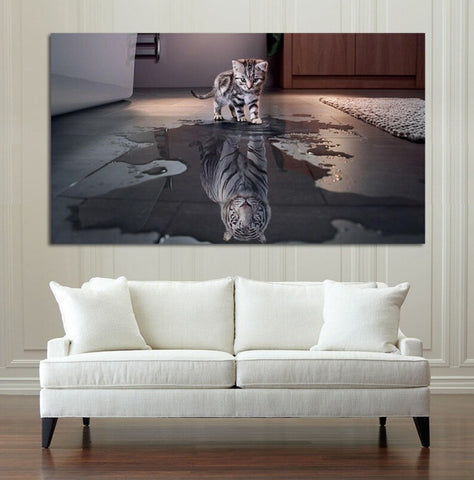The picture showcases a modern living room with a clean, minimalist design. Dominating the foreground is a sleek white sofa adorned with two matching white pillows and supported by dark black legs. The floor beneath the sofa is a rich brown, adding a touch of warmth to the scene. A prominent white paneled wall serves as the backdrop, featuring a striking framed digital artwork. This artwork depicts a gray-white kitten gazing into a puddle, its reflection transforming into a majestic white tiger. The setting within the artwork suggests a bathroom scene, complete with a bath rug, adjacent cabinets, and what appears to be a tub. The juxtaposition of the real and digital elements creates a thought-provoking ambiance, blending everyday simplicity with imaginative storytelling.